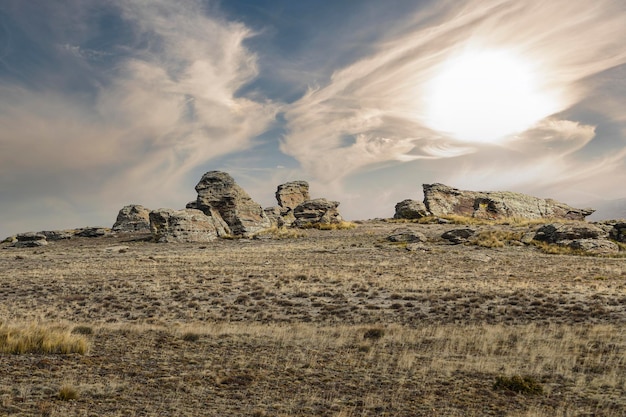The image showcases a desolate hill in a desert-like environment characterized by light gray dirt and interspersed patches of dead, tan grass. Atop the hill, there are several large, chunky rocks with varying shapes; some are elongated and rectangularly horizontal, while others stand tall, boasting either rounded edges or jagged points. These rocks predominantly exhibit gray hues with light tan streaks. The scattered bushes on the hill feature a greenish-yellow tinge, adding sparse hints of color to the otherwise muted landscape. The sky above is a mix of blue and gray, dominated by wispy, wind-swept clouds, suggesting a breezy day. To the right, the bright sun peers through, casting a harsh light over the scene. In the distance, faint mountain-like formations, resembling boulders, loom far back, contributing to the rugged and lifeless atmosphere of the image. The foreground is littered with rocks and dirt, reinforcing the barren quality of this stark, uninhabited terrain.